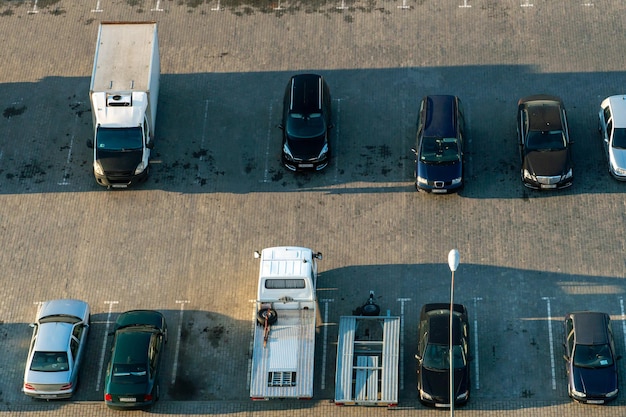The image is a detailed, full-color aerial view of a gray concrete parking lot taken during the daytime with natural light. The photograph is essentially square and taken from several stories above, showcasing two main rows of parked vehicles with the faint presence of a third row at the top, characterized by white lines marking empty spaces. The top row, though partially obscured, includes a large white truck on the left, followed by an alternating pattern of empty spaces and smaller black and blue vehicles, culminating in a white car on the far right. Below this row is a lane of gray concrete. The second row features more vehicles: from left to right, it starts with a white car, then a green car, an empty space, a white truck with a flatbed trailer, another flatbed trailer without a vehicle, a black car, and on the far right, a small silver car. Shadows cast over both rows of vehicles indicate swatches of shade. A street lamp rises from the bottom right corner of the image, adding a vertical element to the otherwise horizontal lines of parked cars and dividing lanes.